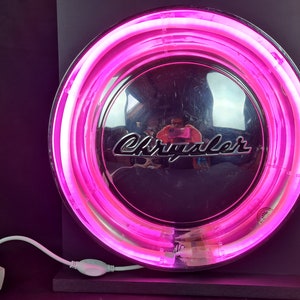This detailed photograph showcases a close-up of a circular, pink neon sign that prominently features the word "Kreisler" or possibly "Chrysler" in a black, italic font at its center. The pink neon tubes encircle the text, giving it an almost hubcap-like appearance. The sign is encased in a lucite container and rests on a gray shelf against a dark background. A white electrical cord extends from the bottom left side of the sign, equipped with an on-off switch. The image also captures reflections within the neon sign, including faint outlines of a person, a bridge, and snippets of the sky, adding depth and intrigue to the composition. The photograph has a central focus but slightly cuts off the right edge of the neon sign.